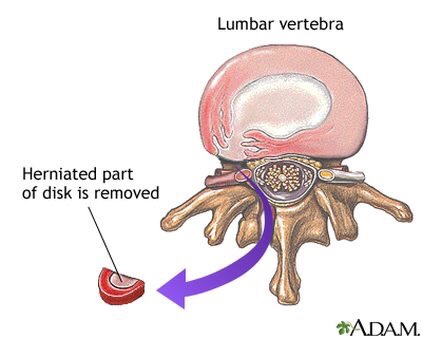This detailed medical illustration features a color drawing of the lumbar vertebrae, highlighting anatomical structures in a cross-sectional view. At the very top, bold black letters label the lumbar vertebra. Below this, there's an image showcasing various anatomical components: a rounded, darker pink structure with a lighter pink interior, an adjacent pink tube on the left, a centrally located silver-gray oval shape containing brown material, and to the right, a silver tube filled with yellow content. Further down, brown branch-like structures resembling tree branches are visible. A prominent purple arrow points to the left, indicating a red, semicircular object. This red shape features a red ring and a lighter pink center, and is labeled with text that reads "herniated part of disc is removed." The background of the image is white, emphasizing the brown-colored vertebra. The annulus fibrosus is depicted in shades of pink and white, and the enlarged cross-section of the herniated disc stands out in red. At the bottom-right corner, there is a logo of a green plant alongside the name "Adam," adding a distinctive detail to the illustration.